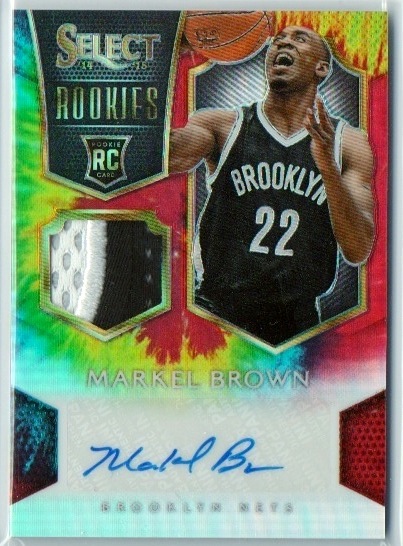This full-color rookie trading card from Select Rookies features Markel Brown, who played for the Brooklyn Nets and wore the number 22 jersey. The portrait-oriented image showcases an African-American man, depicted from the waist up, wearing a black jersey with white text reading "Brooklyn 22". Brown is captured mid-action, looking upwards with his mouth open, seemingly preparing to catch a basketball. The background of the card is a vibrant tie-dye splatter of red, yellow, green, blue, and white. In the upper left corner, there's a banner stating "Select 14 15 Rookies R.C.," while the upper right corner features an image of Brown. Below this, his name, "Markel Brown," is displayed in white text, with his signature in blue ink just beneath it. Accompanying the signature are two geometric shapes: a red four-sided figure to the right and a blue-sided figure to the left, bordered with contrasting colors.